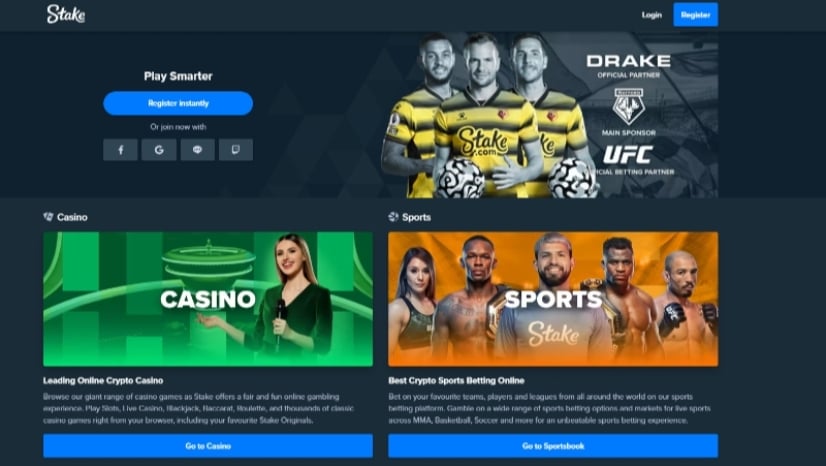This image depicts a betting website with a dark, black background predominantly featuring white text. At the very top, bold white letters spell out "Stake." Adjacent to this is the option to switch languages, with "English" displayed, and a small blue button labeled "Register."

Immediately beneath this header is a rectangular section with white text that reads "Play smarter," accompanied by a blue button. Although the button's full text is unclear, it likely says something akin to "Register Instantly." Below this, there are small square icons representing different sign-up methods: a blue "F" for Facebook, a red "G" for Google, a text messaging icon in grey, and an email icon depicted as a square with a torn paper edge.

In the central image, three men are holding a black-and-white soccer ball. They are sporting yellow and black striped shirts that say "Stake" in black letters. To the right of this image are the words "Drake" and "UFC."

Further down, there are two additional images. The left image features a woman wearing a green, three-quarter sleeve V-neck top. She has dark hair and a light complexion and is holding a microphone. The word "Casino" is overlaid on this image.

On the right side, there is a group of five people. The woman on the left is in a black tank top, with dark hair and is notably attractive. Next to her is a muscular, brown-skinned man who appears to be a boxer; he is shirtless, tall, with a close haircut and clean-shaven. Beside him stands a white man in a blue t-shirt, with a full beard and brownish-blonde hair, smiling. The text "Sports Day" is overlaid on him. Next is another black man, larger and darker-skinned than the first, with a mostly clean-shaven face and a flat-top haircut. The final person is an older boxer with a bald head, who could be white or Hispanic.